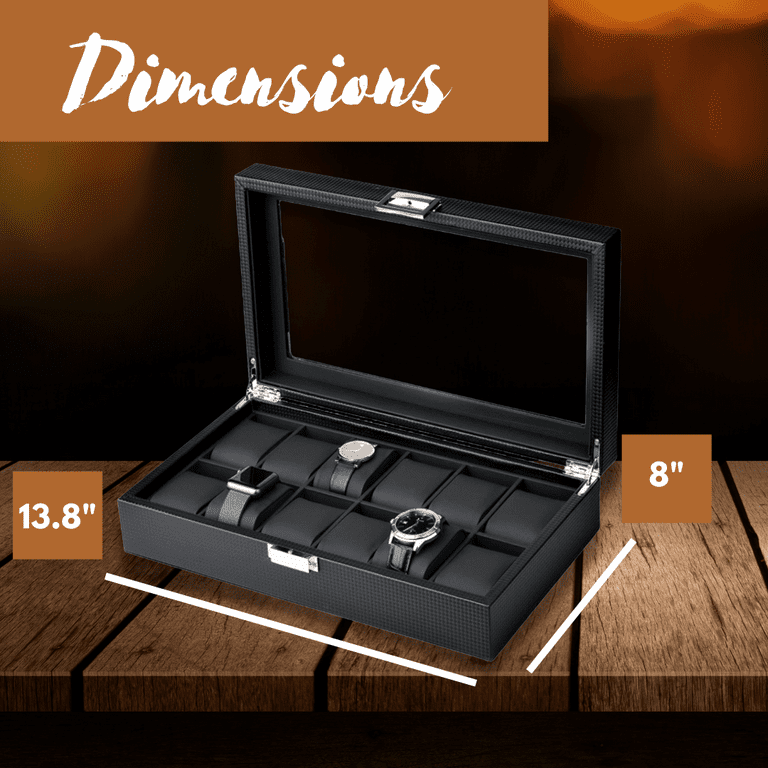This photograph features an open black leather watch case with chrome hardware, including sturdy hinges and a heavy-duty latch at the front. The case contains three watches and has a mirror on the inside, offering a sleek and elegant storage solution. The dimensions of the case are prominently displayed as "13.8 inches wide and 8 inches deep" in white cursive text on a brown rectangular box at the top of the image. The background of the photograph is primarily brown, with varying shades and glares of light, particularly noticeable in the upper right corner. The case itself is placed on a natural wood table or ledge with a prominent grain, consisting of vertically oriented planks that are medium brown in color. The overall setup creates a refined and organized aesthetic, ideal for showcasing watch storage in a stylish manner.